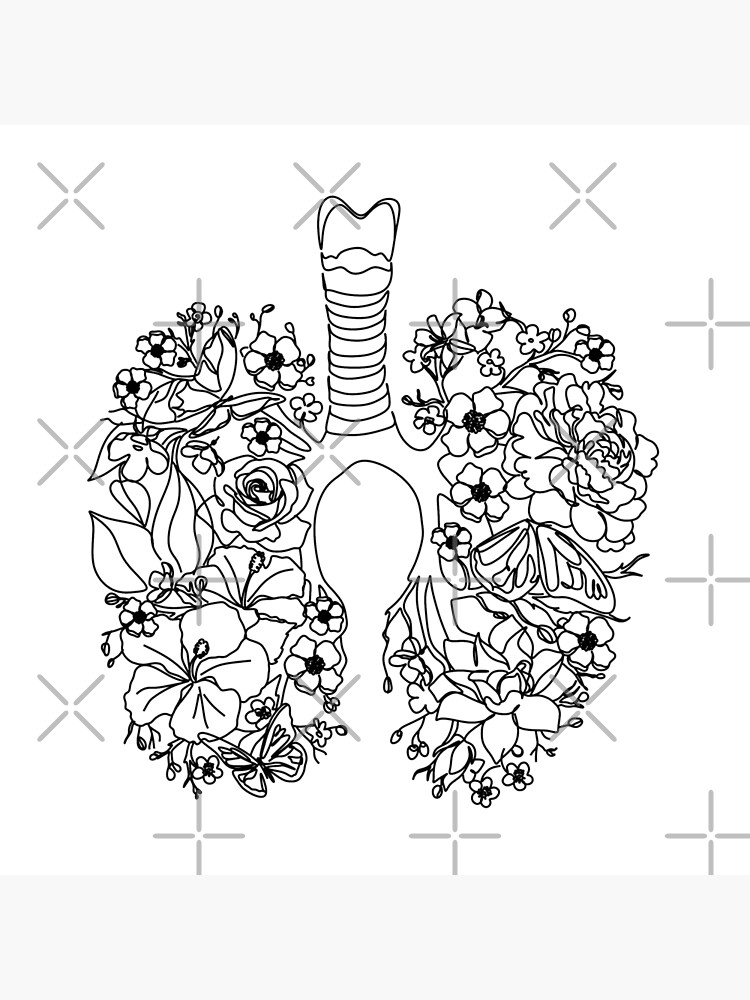The image is a detailed black-and-white ink drawing reminiscent of a paint-by-numbers coloring book. It depicts an artistic rendering of human lungs, with the two lobes represented by an intricate arrangement of flowers and leaves of various shapes and sizes. Among the floral designs, butterflies are interspersed, enhancing the decorative complexity. The lobes are connected by a central windpipe, drawing a parallel to the esophagus and trachea, which is detached from any body and topped with a wavy line. Light gray crosshairs span the white background, suggesting it is intended for coloring, making it suitable for both children’s coloring books and digital fill-in-the-color apps.